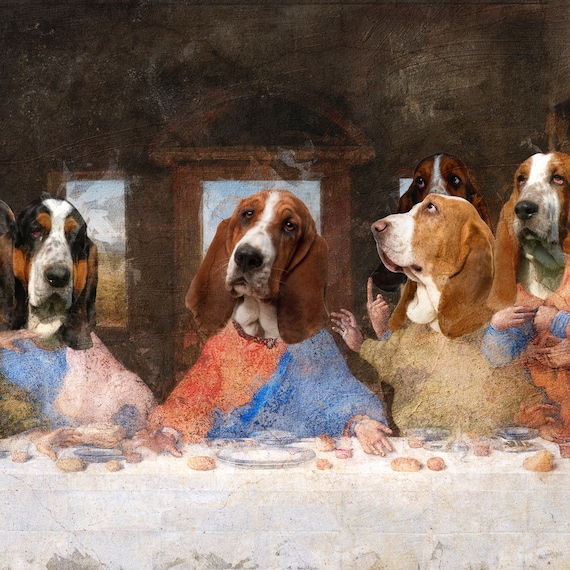The image is a humorous and modified take on the famous painting "The Last Supper," featuring Basset Hounds instead of people. This parody artwork displays a square composition where Basset Hounds are seated at a long table draped with a white cloth, similar to the original painting. Behind the table, there are windows and a ceiling overhead. The central Basset Hound, positioned where Jesus would be, has dark brown ears, fur around its eyes, and is clad in a red and blue tunic. On its left, another Basset Hound wears a pink and blue tunic, with a white face and dark brown to black ears. To the right of the central figure, a light brown Basset Hound donning a yellow tunic is noticeable, characterized by a white snout. Two additional Basset Hounds are positioned behind this dog. The Basset Hounds' heads are real photos of the dogs, all featuring white markings on their faces and chins, with varying colors from chocolate brown to tan and black. The scene is completed with colors such as orange, blue, beige, brown, white, black, gray, dark brown, and pink, making it an engaging blend of classical art style and playful imagery.